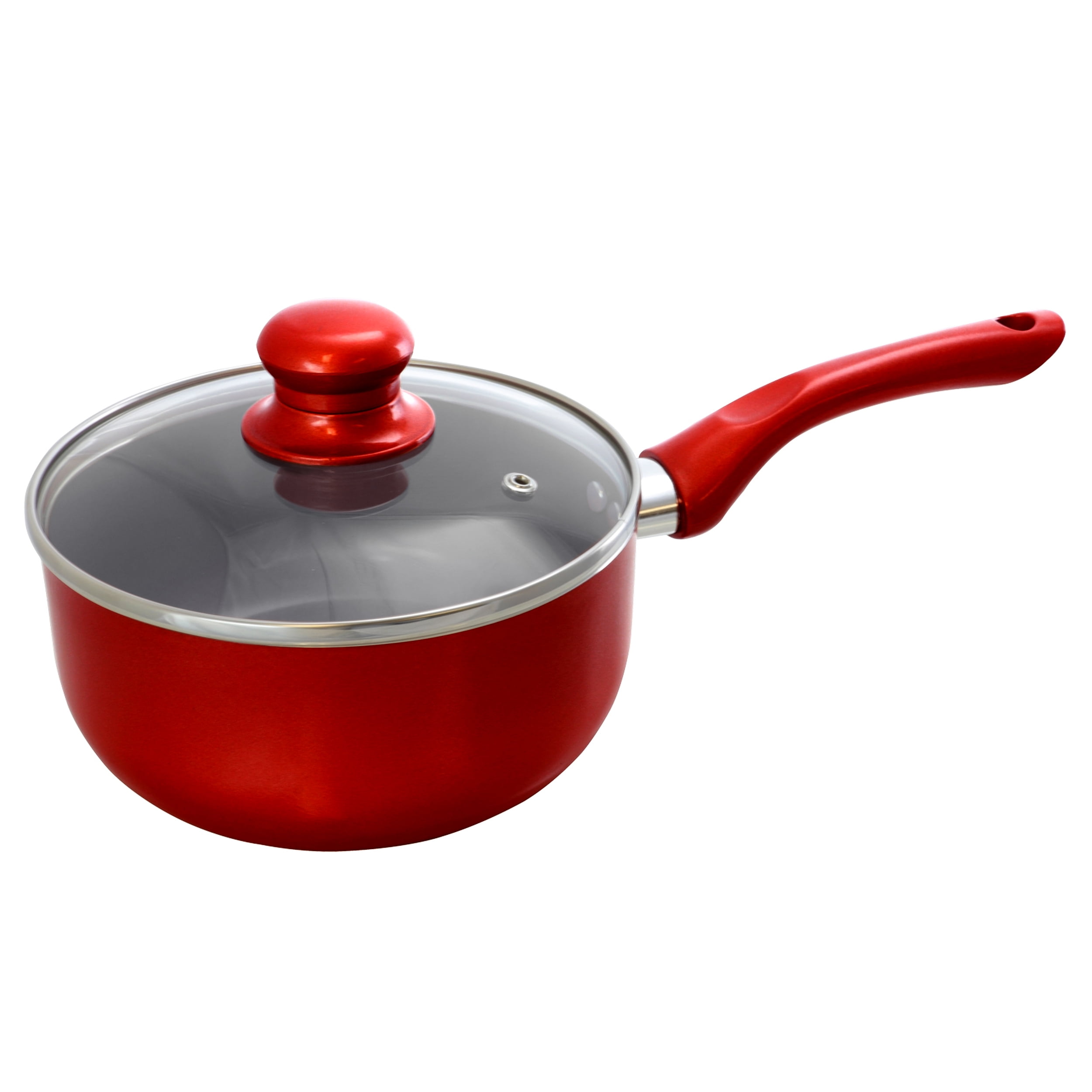The image depicts a small, possibly one-quart-sized cooking pot, ideal for simmering. The pot is round with a red enamel-coated exterior and a matching long handle, which features a hole for hanging. The handle is attached to the pot with silver rivets. The clear glass lid has a vent hole and a circular, doorknob-like handle, also in the same bright cherry red as the pot and its handle. The interior of the pot is a dark, non-stick surface, likely black or dark gray. Positioned against a white background, the pot is perfectly in focus and well-lit, with no other objects or text present, making it look like a professional advertisement photo.